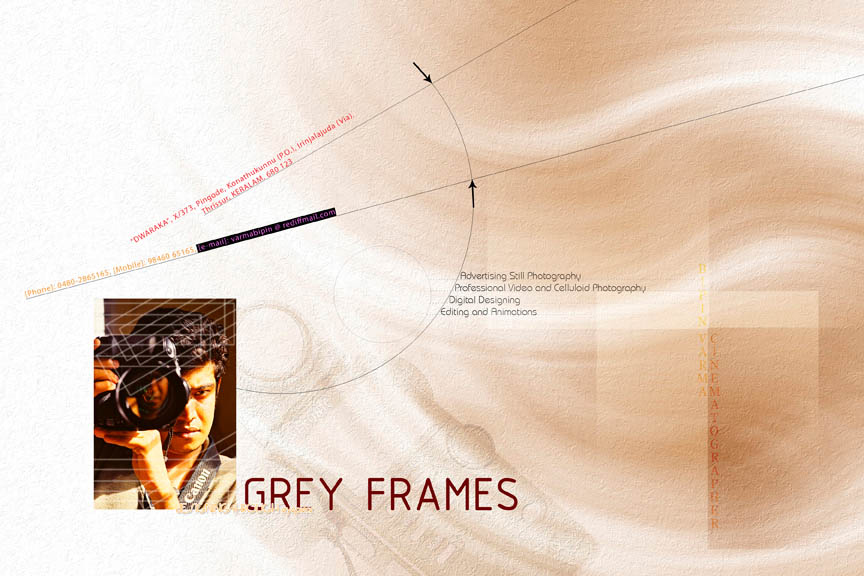In the lower-left corner of the advertisement, a young man of likely Indian, Pakistani, or Middle Eastern descent with dark skin and jet-black hair is shown holding a large camera up to his eye, obscuring one of his eyes. Visible in the camera lens is the faint image of a girl's face, presumably the subject he is photographing. The backdrop consists of a brownish, board-like texture, giving the entire image a warm, beige tone. The advertisement prominently features the name "Grey Frames" at the bottom in large text. Surrounding this central image are details of the services offered, including still photography, professional video, celluloid photography, digital designing, editing, and animations. The English text providing these details is written in grey, suggesting a promotional piece for the photographer's business named Grey Frames.